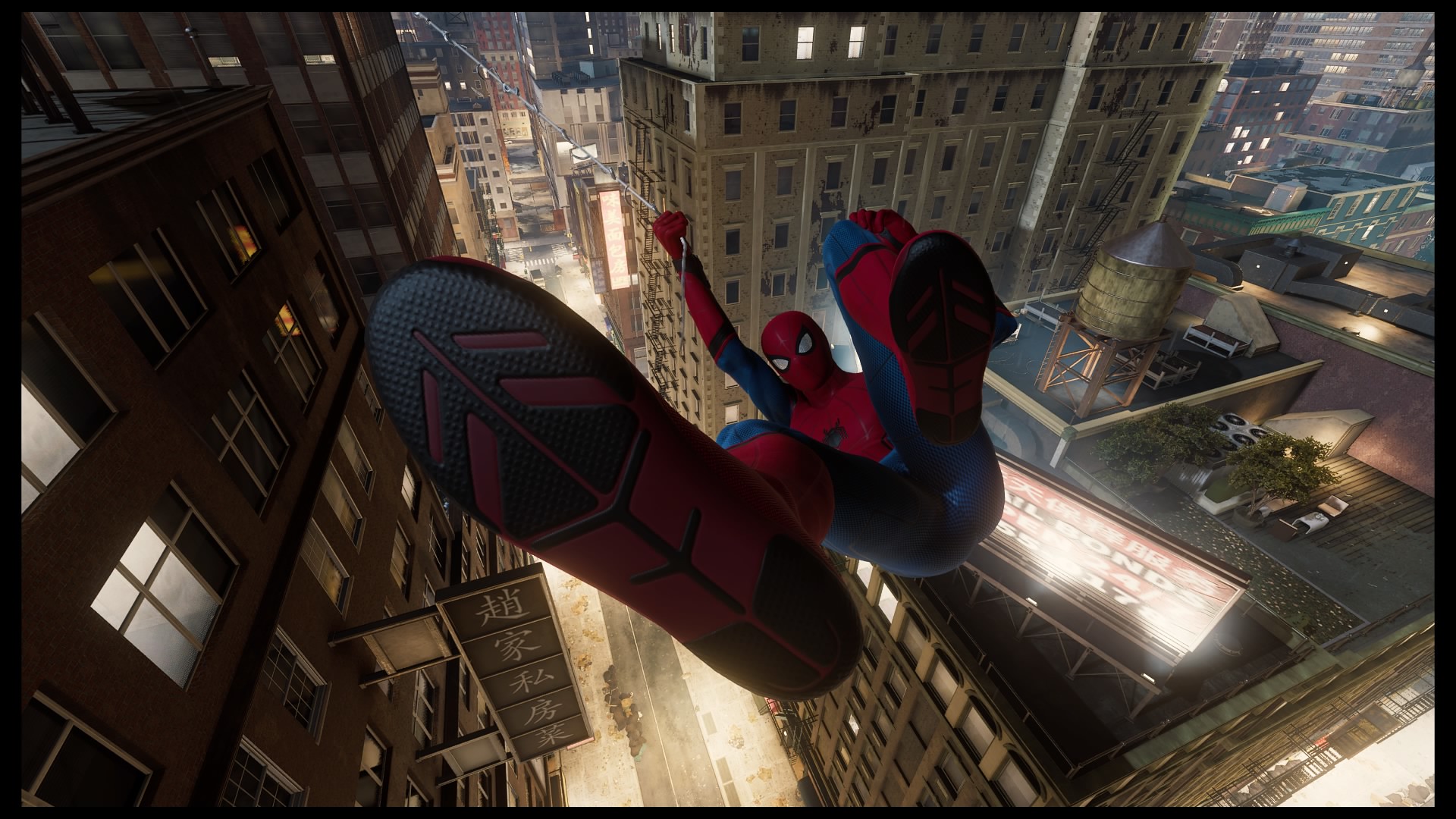The image is a detailed screenshot from a Spider-Man movie or video game. It showcases Spider-Man swinging high above a densely packed cityscape at night. The scene captures him mid-jump, holding onto a spider web strand with his right hand that extends from the top left corner. The perspective is from below, emphasizing the underside of his right shoe, which is black with red accents, prominently in the foreground. His left leg is bent at the knee, revealing the black sole of his shoe. Spider-Man's iconic suit is visible, and his face is turned towards the camera as he appears to be flying through the air. The entire backdrop consists of towering buildings, with a street scene faintly visible far below, suggesting a great height. Specific details include a sign with Chinese characters on a building to the left and a lit billboard with a small rest area and a water tower on top of a building to the right. The image is framed with a black border, reminiscent of a video still.